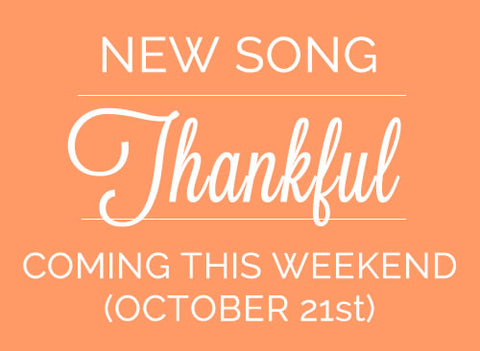The image is a rectangular, computer-generated advertisement banner with a solid orange background. It prominently features white text, announcing a new song release. At the very top, in white capital letters and underlined, it reads "NEW SONG." Beneath this, centrally placed, is the song title "Thankful," rendered in bold, white script and also underlined. At the bottom of the image, in white capital letters, the text announces "COMING THIS WEEKEND," with the release date "October 21st" following in parentheses. The layout is simple yet well-spaced, giving the impression of a billboard advertisement or a social media announcement slide, characterized by its limited color palette of orange and white.